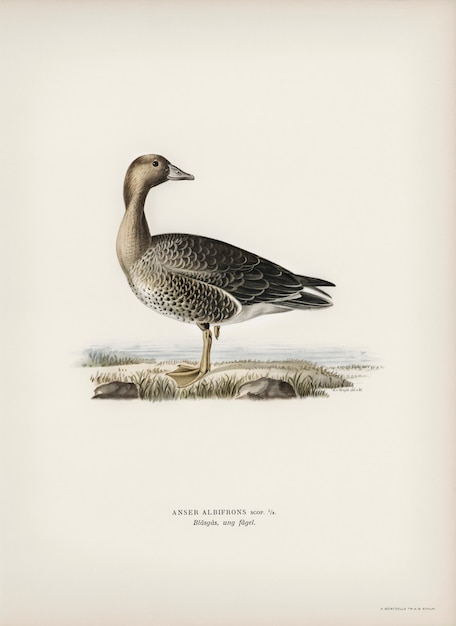This detailed image appears to be a page from a book, depicting a bird that resembles a duck, possibly a water bird, rendered in a style reminiscent of Audubon. The bird, predominantly brown with a gradient of lighter brown and white feathers, stands on a small piece of land next to a few rocks with sparse brush. Its body faces left while its neck twists backward, making its head face the right. Beyond the bird, there's a hint of blue water, suggesting the bird is near a shore. The background is primarily beige, providing a simplistic yet detailed contrast to the intricate drawing. At the bottom of the image, in small capitalized text, it reads "ANSWER ALBIFRONS," followed by some illegible text.